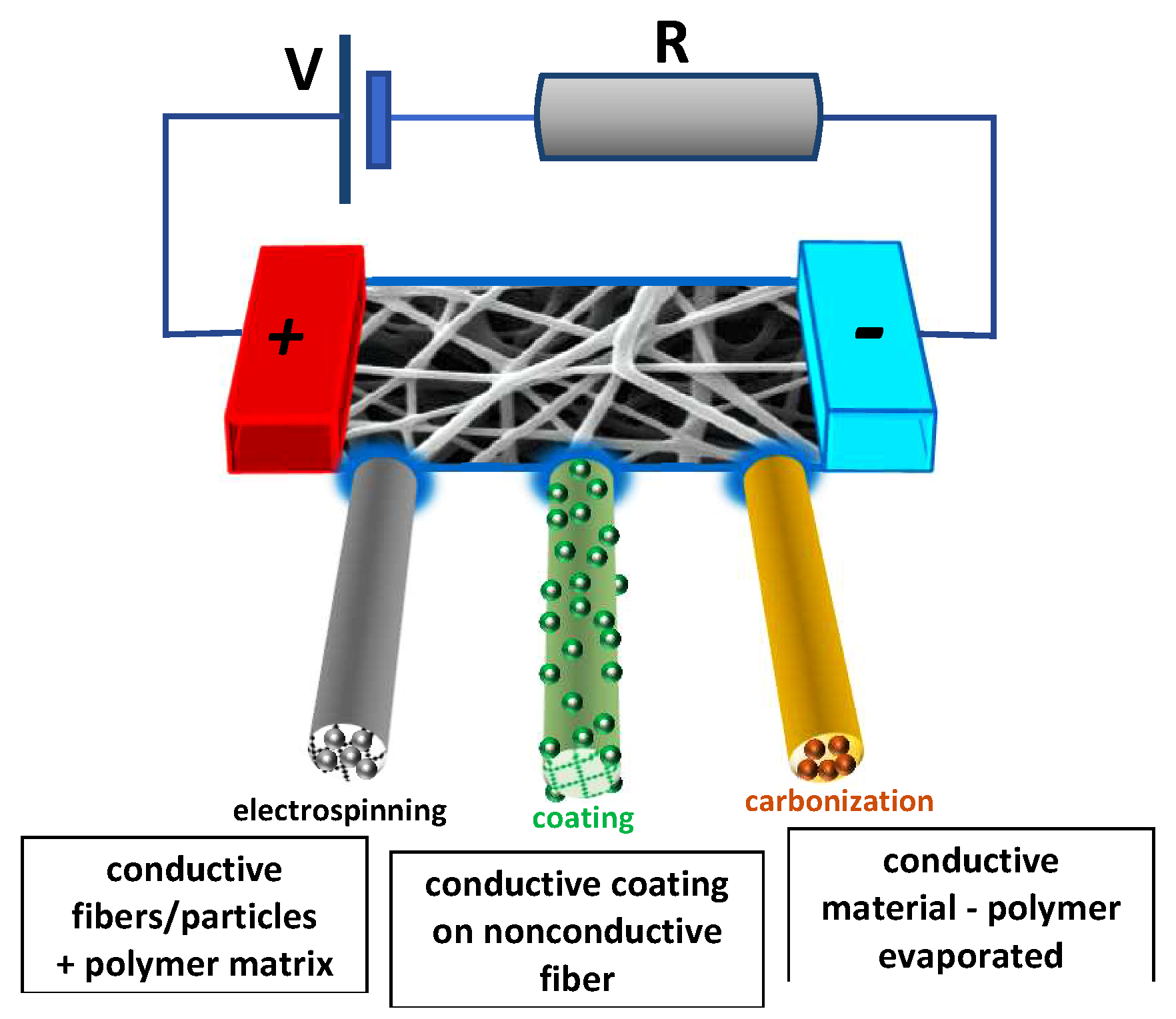The diagram is a detailed, scientific schematic presented in a horizontal, rectangular layout with a blue-bordered white background. On the far left, there's a vertical dark blue line beside an uppercase "V". Next to this is a vertically oriented dark blue-outlined rectangle with a light blue center that aligns with a black capital "R" enclosed in a gray, blue-bordered rectangle. Below, there is a sequence of labeled rectangular sections with thin black borders. The leftmost section reads "Conductive fibers/particles + polymer matrix," followed by "Conductive coating on non-conductive fiber," and "Conductive material, polymer evaporated." Above these sections, from left to right, the labels "Electrospinning," "Coating," and "Carbonization" correspond to silver, green-coated, and gold/orange rods respectively. A red plus sign is depicted on the left of the gold/orange rods, with a turquoise rectangle and a blue outlined minus sign on the right. White strands are stretched between the positive and negative symbols. A connecting line from the plus sign ascends to the "V" while another line from the minus sign ascends to the "R," illustrating an electric pathway.